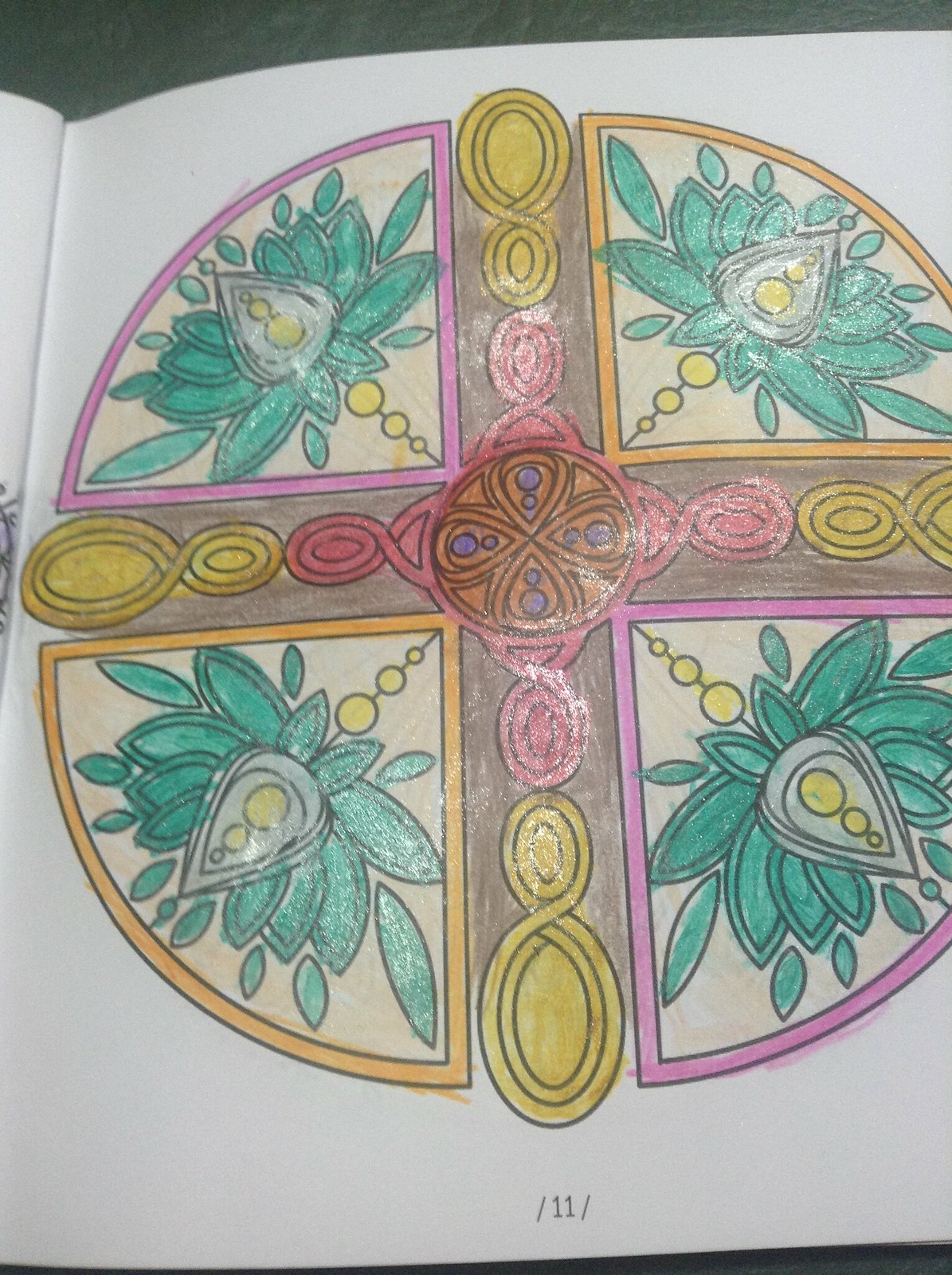The image is a zoomed-in photograph of a page from a Christian-themed coloring book, most likely intended for children, possibly used in a Sunday school setting. The focal point of the page, labeled as "Page 11," features an intricately designed cross formed by interlocking ovals and pie-shaped segments. The cross is surrounded by a variety of vibrant colors, including red, orange, yellow, green, and pink, likely applied with crayons. Each of the four pie-shaped sections contains a green floral pattern with yellow bulbs, outlined in pink and orange, all set against a white backdrop. The detailed and colorful elements suggest it is a page meant to engage and entertain children through creative coloring.